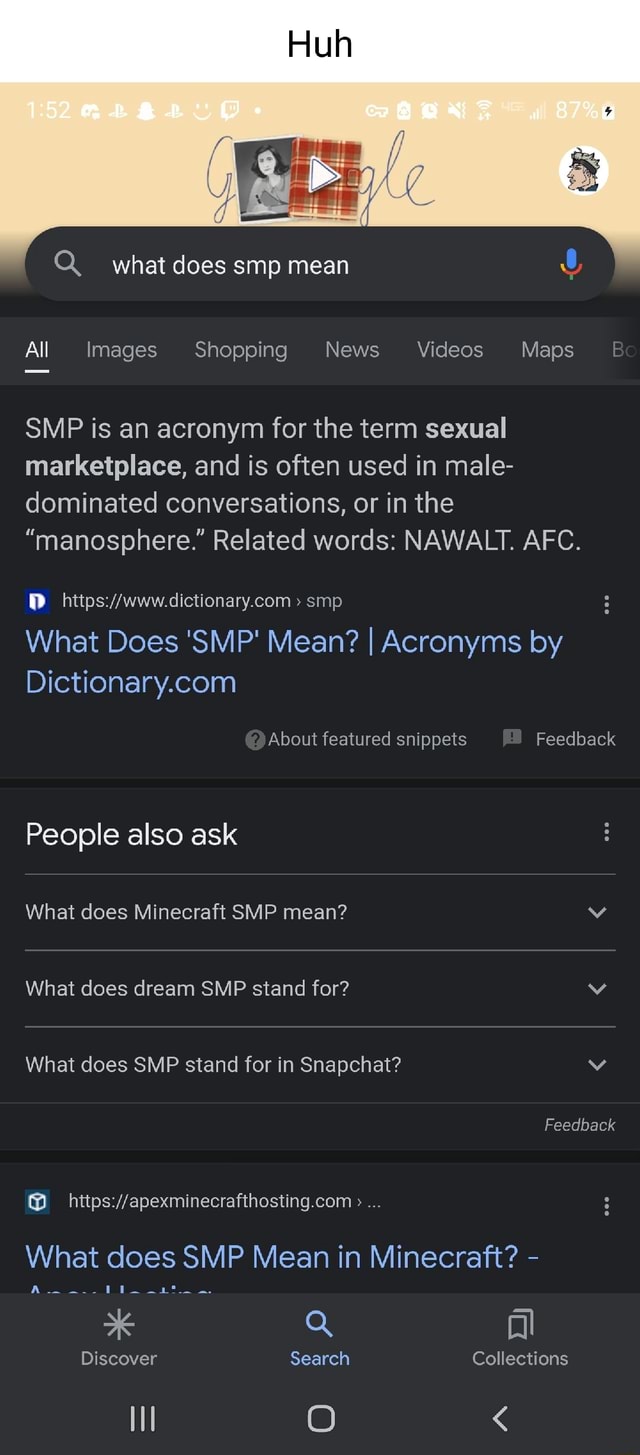A mobile screenshot captures a Google search page with a special Google Doodle, featuring a stylized illustration of a woman accompanied by French text and a plaid design incorporated into one of the letters. Directly beneath this customized Google logo is the search bar, which contains the query "what does SMP mean". To the left of the search bar, there is a magnifying glass icon, and to the right, a microphone symbol. Below the search bar, navigation tabs are displayed: "All," "Images," "Shopping," "News," "Videos," and "Maps".

The first search result explains that "SMP" is an acronym for "sexual marketplace," a term often used in male-dominated discussions or the "manosphere." It mentions related terms such as "NAWALT" and "AFC," and is linked to dictionary.com under the title "What does SMP mean? Acronyms by dictionary.com". Beneath this, there is a section titled "About featured snippets" and "Feedback".

Following this, a "People also ask" section appears with related questions: "What does Minecraft SMP mean?", "What does Dream SMP stand for?", and "What does SMP stand for in Snapchat?" Each question has an arrow pointing down, indicating expandable answers.

Next, an entry from ApexMinecraftHosting.com is listed, accompanied by three dots for additional options. Below this, an incomplete snippet hints at more information about what SMP means in Minecraft. At the bottom of the screenshot, there is a partially visible prompt for "Discover search collections," showcased with small icons.